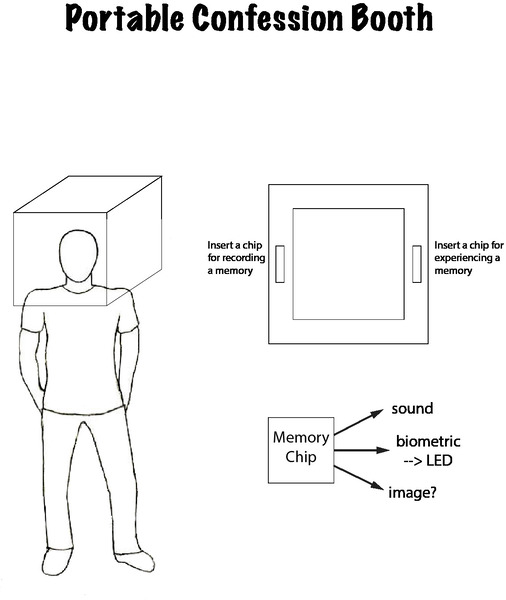This black and white technical sketch depicts a faceless man standing with his hands in his back pockets, wearing a box over his head. The illustration, titled "Portable Confession Booth," seems to brainstorm or outline the concept of a device that allows for memory recording and experiencing. On the right side of the man, the diagram details two slots on the box—one for inserting a chip to record a memory, and another for inserting a chip to experience a memory. Below this, additional information about the memory chip is provided, pointing out capabilities like sound, biometric LED indicators, and image processing. The overall composition suggests a simplified, yet thoughtful technical drawing aimed at illustrating how this device might function in practice.